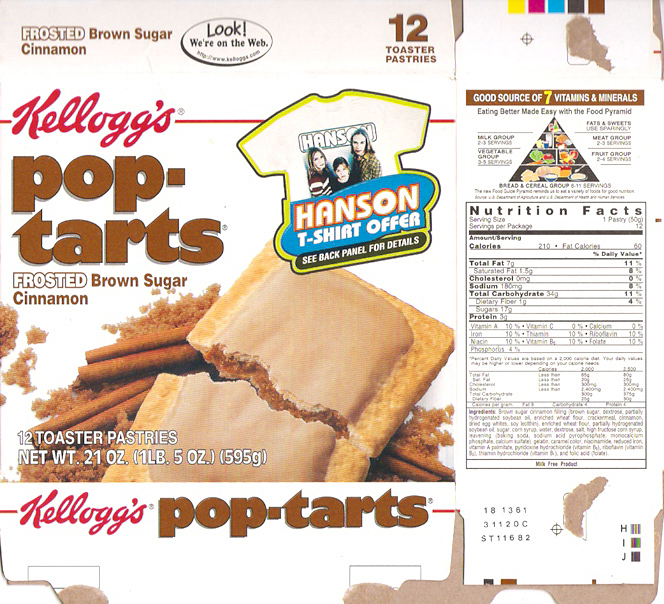This image features a flattened, empty box of Kellogg's Pop-Tarts, specifically the Frosted Brown Sugar Cinnamon flavor. The box is laid out to display both the front and side panels. Prominently on the front, the flavor is highlighted with text and an appetizing photo of an iced brown sugar Pop-Tart broken in half, revealing its filling. Surrounding the broken Pop-Tart are cinnamon sticks and a dusting of ground cinnamon, all set against a clean, white background. The side panel of the box shows the nutrition facts label, and at the top, there's an image of the food pyramid accompanied by the text, "Eating better made easy with the food pyramid."